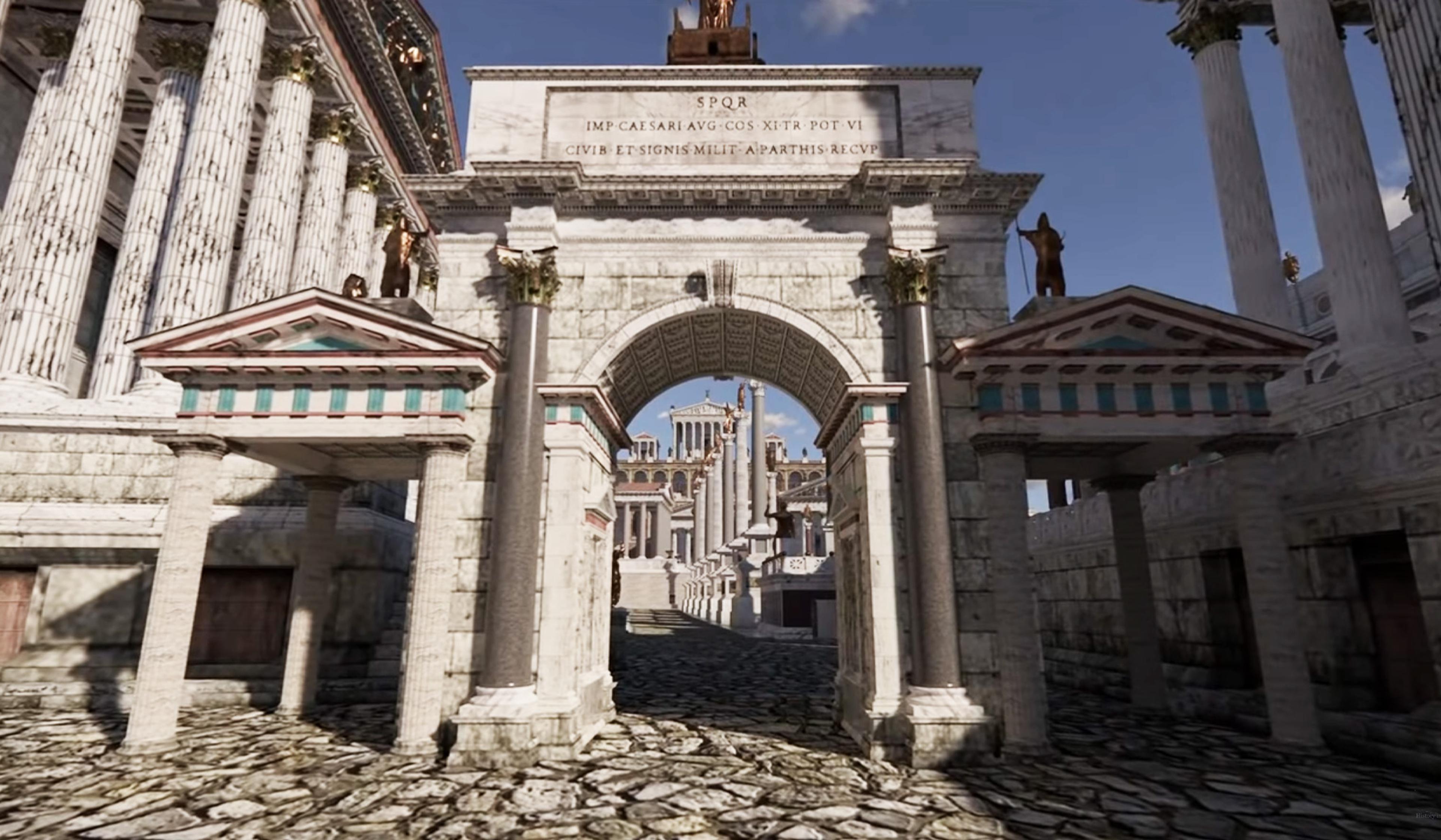This color photograph depicts an ancient Roman or Greek architectural site under a clear blue sky. The image is dominated by a grand archway situated centrally, flanked by tall, imposing concrete columns. The archway, inscribed with Latin text, has partially cut-off metallic sculptures on top. On either side of this archway are smaller, identical covered areas with teal accents near the roof. In the left portion of the image, additional columns support the roof of a large building. The ground is made of cobblestone, extending towards the background, which reveals more columns and grand stone buildings adorned with human-figure statues. The clear midday lighting enhances the strikingly white stone structures, emphasizing their ancient, historic beauty.